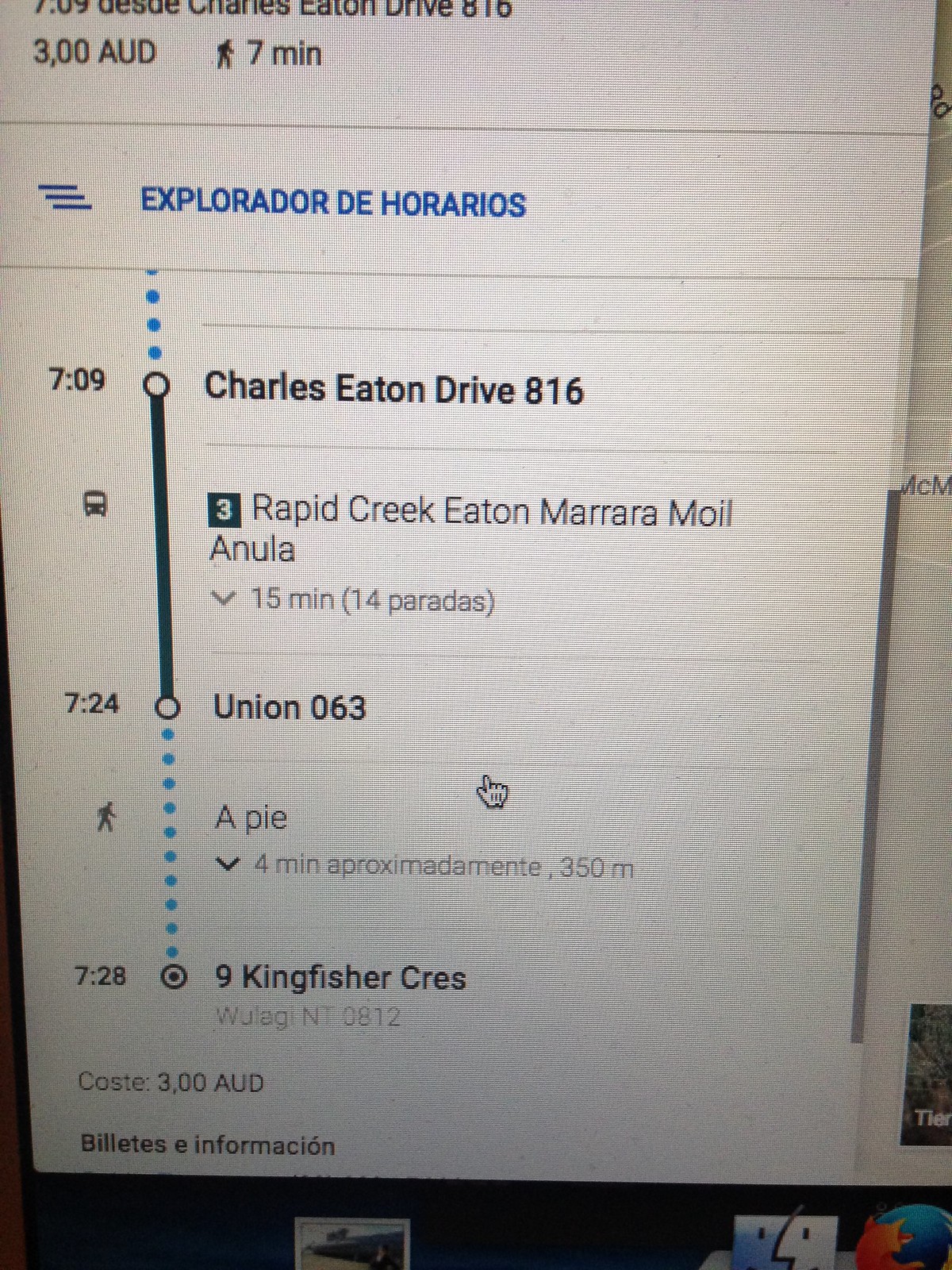A computer screen displaying a Google Maps interface in Spanish is showing detailed directions to a specific location. The journey begins at Charles Eaton Drive, 816, and involves taking a bus to Union 063. After getting off the bus, there is a 4-minute walk to 9 Kingfisher Crest. The entire trip includes a brief 7-minute walk at the beginning and costs 3 AUD. The text is primarily in Spanish, providing clear instructions and costs associated with the route.